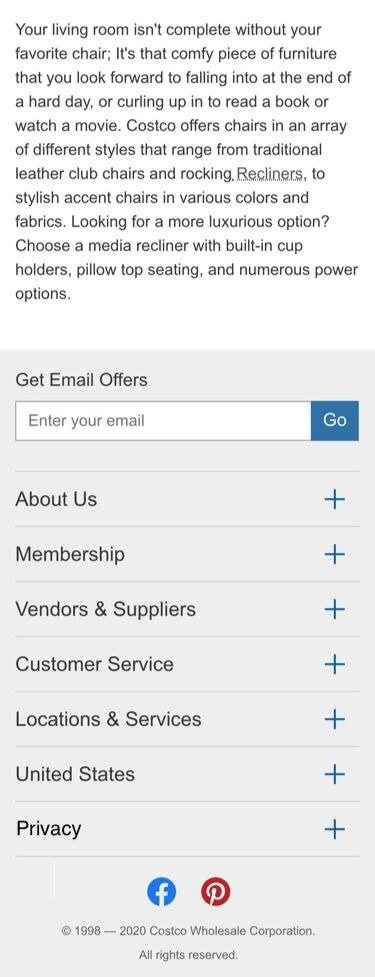In this image, a promotional text from Costco emphasizes the importance of having a favorite chair in your living room. The text highlights the comfort and relaxation that a well-chosen chair can provide after a long day, whether for lounging, reading a book, or watching a movie. Costco offers a wide selection of chairs, including traditional leather club chairs, rocking recliners, and stylish accent chairs available in various colors and fabrics. For those seeking a more luxurious option, the text suggests media recliners equipped with built-in cupholders, pillow-top seating, and numerous power features. Additional options are provided at the bottom for email offers, with links for smarter shopping connections, more information about the company, membership details, vendor and supplier information, customer service assistance, and locations and services. The text also references privacy details specific to the United States.